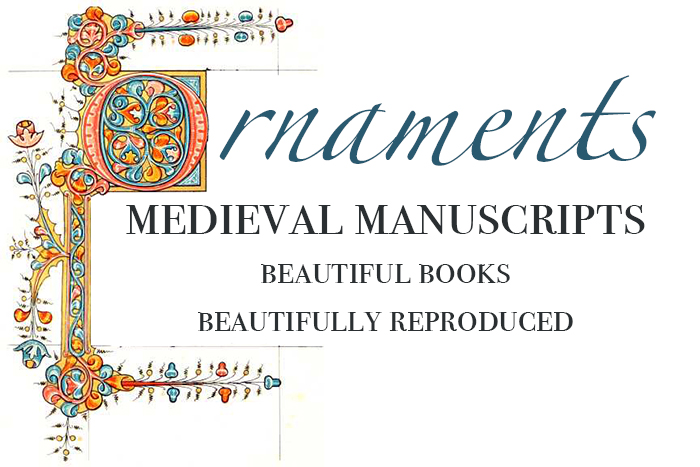This image appears to be a cover for a medieval design book set against a white background. Prominently featured is the word "Ornaments," written in a peculiar blue font with a distinctive, flowery "O" that looks like a plant. The ornamental "O," intricately designed in blue, orange, yellow, and red, connects seamlessly with the border of the design. Below "Ornaments," the phrases "Medieval Manuscripts," "Beautiful Books," and "Beautifully Reproduced" are displayed in a bold black, all-caps font, arranged in three centered lines. Adding to the medieval aesthetic, a yellow, blue, and orange floral scroll design is situated to the left of the text. The layout is horizontal, featuring lines at the top and bottom of the image, framing the design elements elegantly.